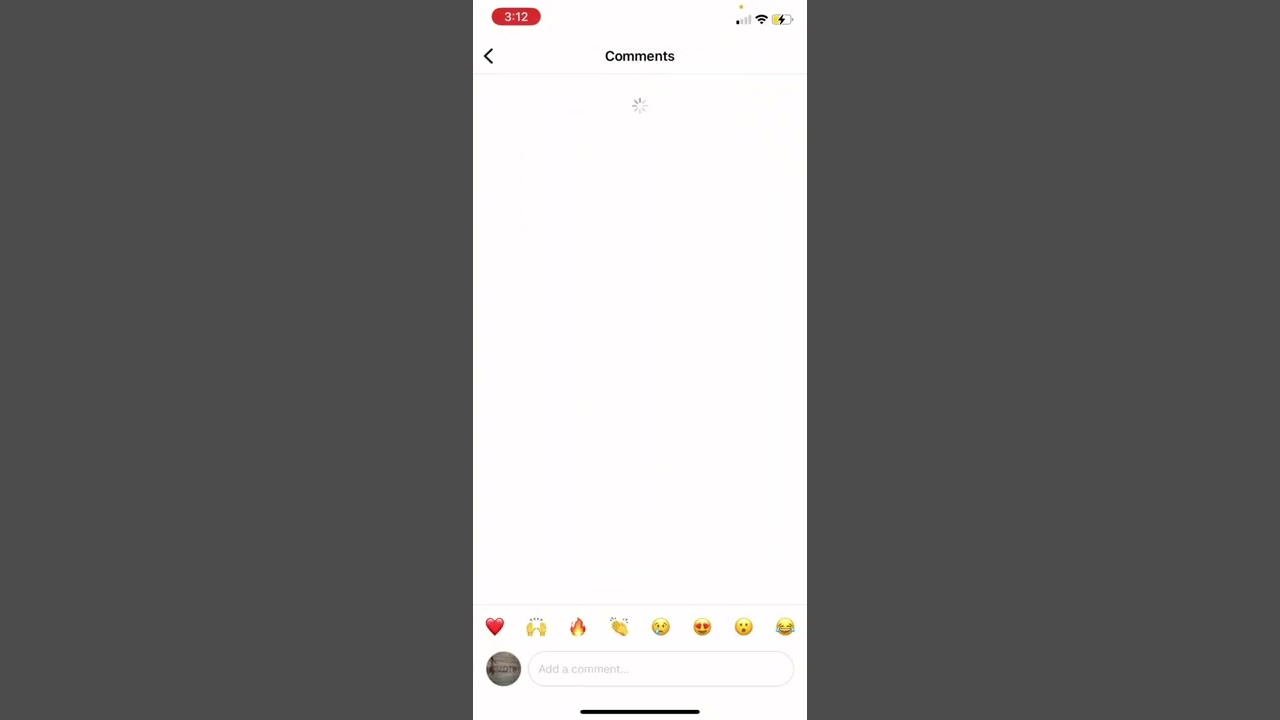The image is a screenshot of a smartphone displaying what appears to be the comments section of an Instagram post. Notably, no actual post is visible, only the comments interface. 

At the top of the screen, the current time is displayed as 3:12, enclosed in a red, pill-shaped box. To the right of the time, the phone displays one bar of cell service, full-strength Wi-Fi connectivity, and a battery icon indicating it is approximately at half capacity and currently charging. 

The predominant color of the screen is white, except for some elements in black. At the very top, the word "Comments" is prominently displayed in black. To the left of this word, there is a back arrow icon. Directly below "Comments," a loading circle is actively spinning, indicating that the comments section may be in the process of refreshing or loading content. As of now, no comments are shown.

At the bottom of the screen, a row of emoji icons is visible, including a heart, two hands held out, a flame, applause, a crying face, a heart-eyes face, a surprised face, and a laughing face. These are likely quick-response icons for the user to react to comments. 

The user’s profile icon, which appears to be a small purple car on a gray background, is located just above this row of emojis. Next to the profile icon, text prompts the user to "Add a comment." 

The screenshot has been taken against a very wide, gray blank background, possibly suggesting that the image is intended for viewing or editing purposes.